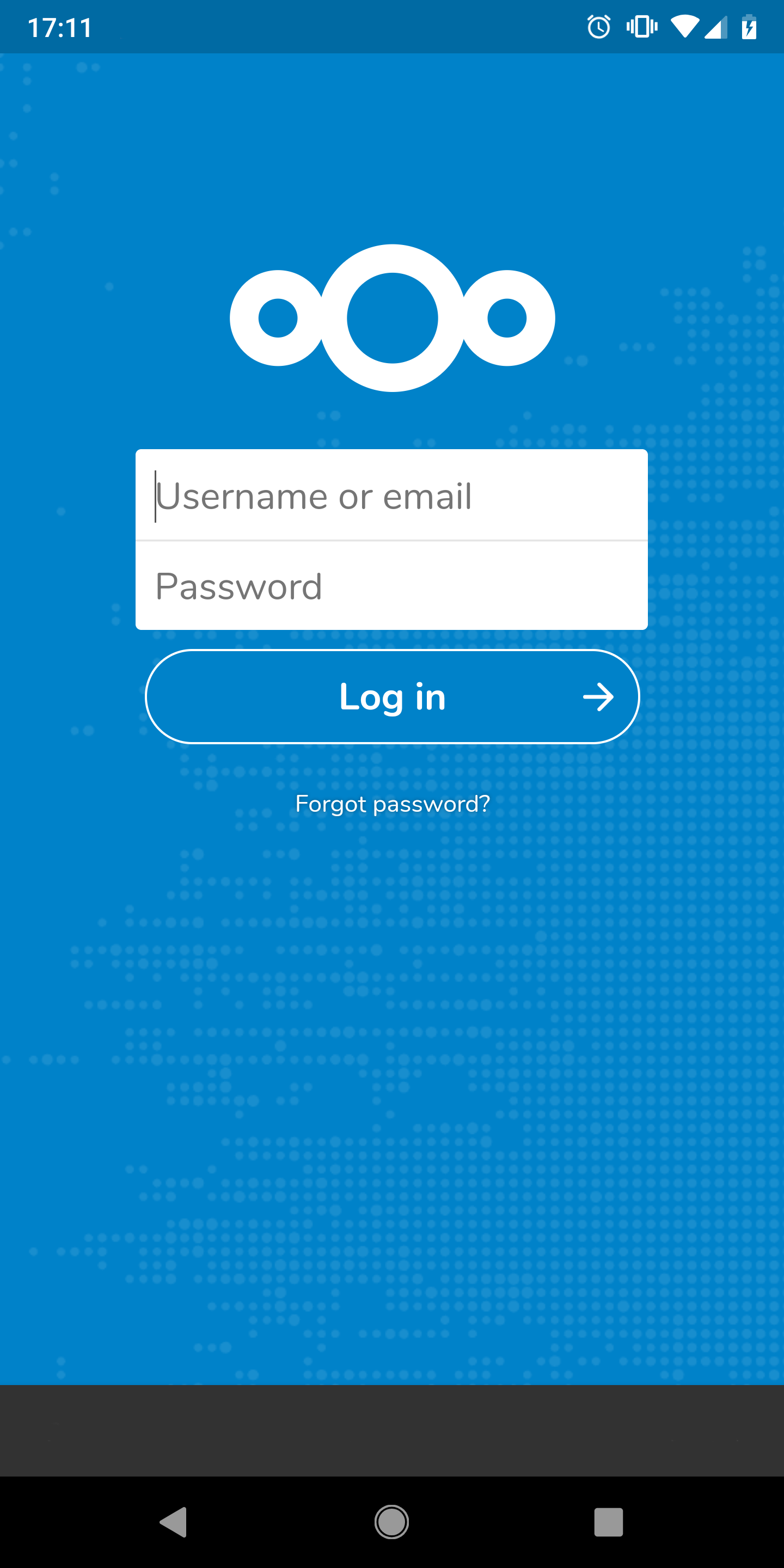This is a detailed login screen from a website, predominantly featuring a blue theme. At the very top of the screen is a dark blue, thin bar. On the left of this bar, it displays the time, "17:11." On the right side of the bar are several computer icons, including a clock, a battery indicator, and other miscellaneous images.

The main part of the screen is a lighter blue color. Centrally located is a white login box with gray font, designed for entering a username or email and a password. Above this login box is a logo consisting of a small white circle, a larger white circle, and another small white circle on the opposite side, all thickly lined.

Below the login fields, there is a white-outlined bar with the word "Login" in white letters. The "L" is capitalized and the following letters "OG IN" are in small letters, separated by a space. Next to "Login" is a white arrow pointing to the right.

Further below the login button are the words "Forgot password?" in white. The "F" in "Forgot" is capitalized, and the rest are in lowercase letters. 

The background continues in blue under this text, transitioning into a gray bar, followed by a black bar at the very bottom. The black bar features three white icons: a left-facing arrow on the left edge, a central circular button, and a square button on the right edge.